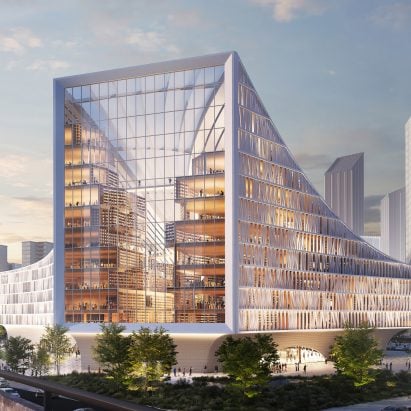The image features a large, futuristic building with a unique architectural design, appearing to have been created using computer graphics. The structure stands prominently with its light gray facade and extensive glass walls that reveal multiple tiers and levels within. One side of the building, likely about 10 stories tall, maintains a rectangular shape, while the opposite side slopes downwards, resembling a ramp, reducing the height to around 5 stories at its lowest point. This gives the building an intriguing, asymmetrical appearance. The surrounding scene shows a blue sky with white clouds, flanked by additional skyscrapers on both the left and right. In the foreground, you can see a lawn with four green trees, some dirt, and a sidewalk. The overall image is somewhat grainy, further emphasizing the digital construction of this architectural marvel.